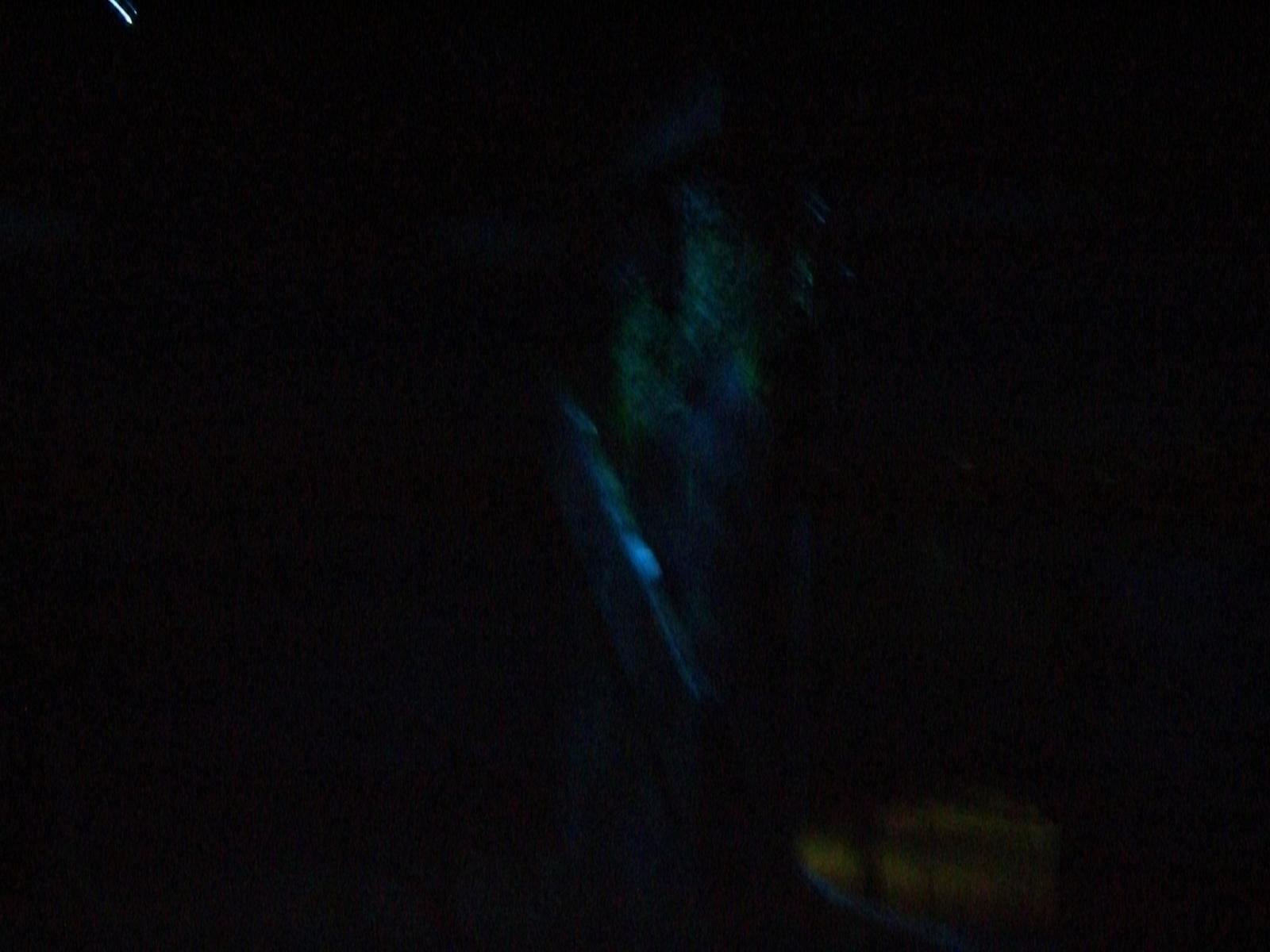The image is predominantly black, with a limited and indistinct lighting that makes it challenging to identify specific details. Centrally positioned is a faint fluorescent streak in light blue, possibly outlining a hand, containing various shades of dark blue, gray, and pastel colors. This central element suggests a medical imaging scan such as an MRI or sonogram. The entire background remains almost entirely pitch black, with just a slight touch of light near the top left corner and a very light green patch toward the lower right. The image is poorly lit and blurry, further complicating efforts to discern whether it depicts an indoor or outdoor scene, rendering the overall scene obscure and resembling a poorly developed photograph.